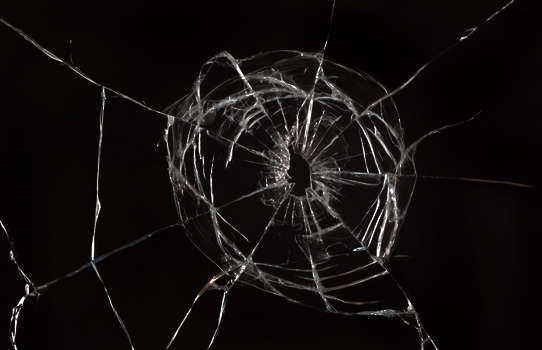The image showcases a close-up of a broken pane of glass against a completely black background, accentuating the dramatic shattering effect. Central to the image is an oblong hole, likely caused by a bullet, surrounded by a series of intricate cracks that emanate outward. The immediate area around the hole features tightly packed, circular cracks, resembling a crystalline or spider web pattern. As these cracks spread outwards, they become broader and more chaotic, extending in various directions and creating a complex network of fissures. The overall effect is a mesmerizing pattern that suggests a powerful impact at the center, with radiating lines that emphasize the force and direction of the break. The stark contrast between the clear, shattered glass and the inky black background heightens the visual impact, making the details of the broken glass appear almost luminous and crystalline.